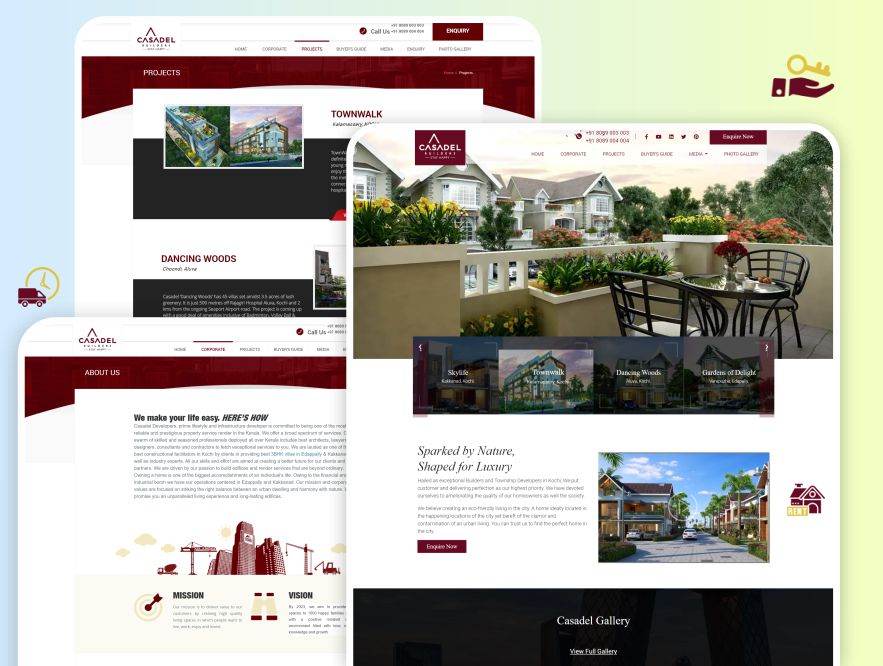The image depicts the homepage of Casadel Builders, a luxury home and corporate project construction company likely based in India, inferred from the visible area code. The website features an organized navigation menu with options including Home, Corporate Projects, Buyer’s Guide, Media, and Photo Gallery, highlighting their diverse range of offerings.

Notably, Casadel Builders specialize in creating high-end residential projects, as evident from project names such as Skylife, Downwalk, and Gardens of Delight, which showcase upscale living environments in India. A prominent section titled "We Make Your Life Easy, Here's How" outlines the company's mission and vision, emphasizing their commitment to excellence and customer-centric approach.

The site also boasts an extensive photo gallery, providing a visual portfolio of completed projects that echo luxury and sophistication. Additionally, the firm appears to prioritize eco-friendly practices, integrating sustainable living principles into their developments. Overall, Casadel Builders present themselves as dedicated luxury and township developers with a focus on quality, comfort, and environmental consciousness.